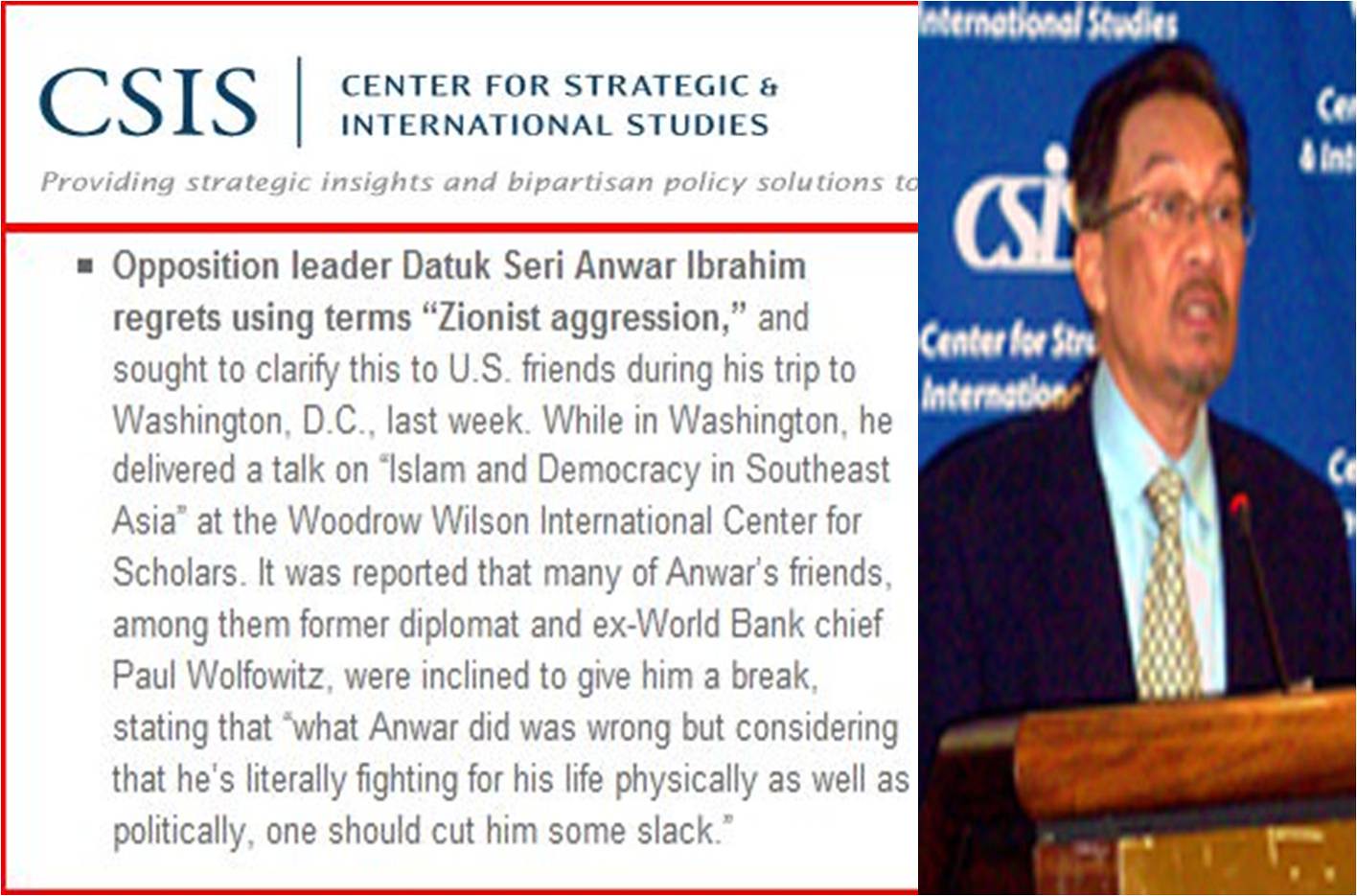The image depicts an article with an inset photograph on the right side extending from top to bottom. The photograph shows a middle-aged Asian man, likely in his 50s, standing behind a brown wooden podium with a microphone. He is facing somewhat three-quarters to the right, adorned in a dark navy suit jacket, light blue shirt, and a tan printed tie with a diamond pleated design. The man has glasses, black hair, and a thin mustache. The background features a dark blue wall with white lettering.

On the left side of the image is the main article outlined in red. The background of the article is white with dark blue or black text. The headline reads "CSIS | CENTER FOR STRATEGIC AND INTERNATIONAL STUDIES" in uppercase. Below this, in italic serif font, it reads "Providing Strategic Insights and Bipartisan Policy Solutions." A horizontal red line separates the headline from the main article. The article starts with a bulleted paragraph, justified to the left, stating:

"Opposition Leader Datuk Seri Anwar Ibrahim regrets using the term 'Zionist aggression' and sought to clarify this to U.S. friends during his trip to Washington, D.C., last week. While in Washington, he delivered a talk on 'Islam and Democracy in Southeast Asia' at the Woodrow Wilson International Center for Scholars. It was reported that many of Anwar's friends, among them former diplomat and ex-World Bank chief Paul Wolfowitz, were inclined to give him a break, stating that 'what Anwar did was wrong, but considering that he’s literally fighting for his life physically as well as politically, one should cut him some slack.'"

The entire image forms a horizontal rectangle with the text to the left and the image of the man at the podium to the right. The colors evident in the image include shades of brown, tan, yellow, gold, blue, black, red, gray, and white.